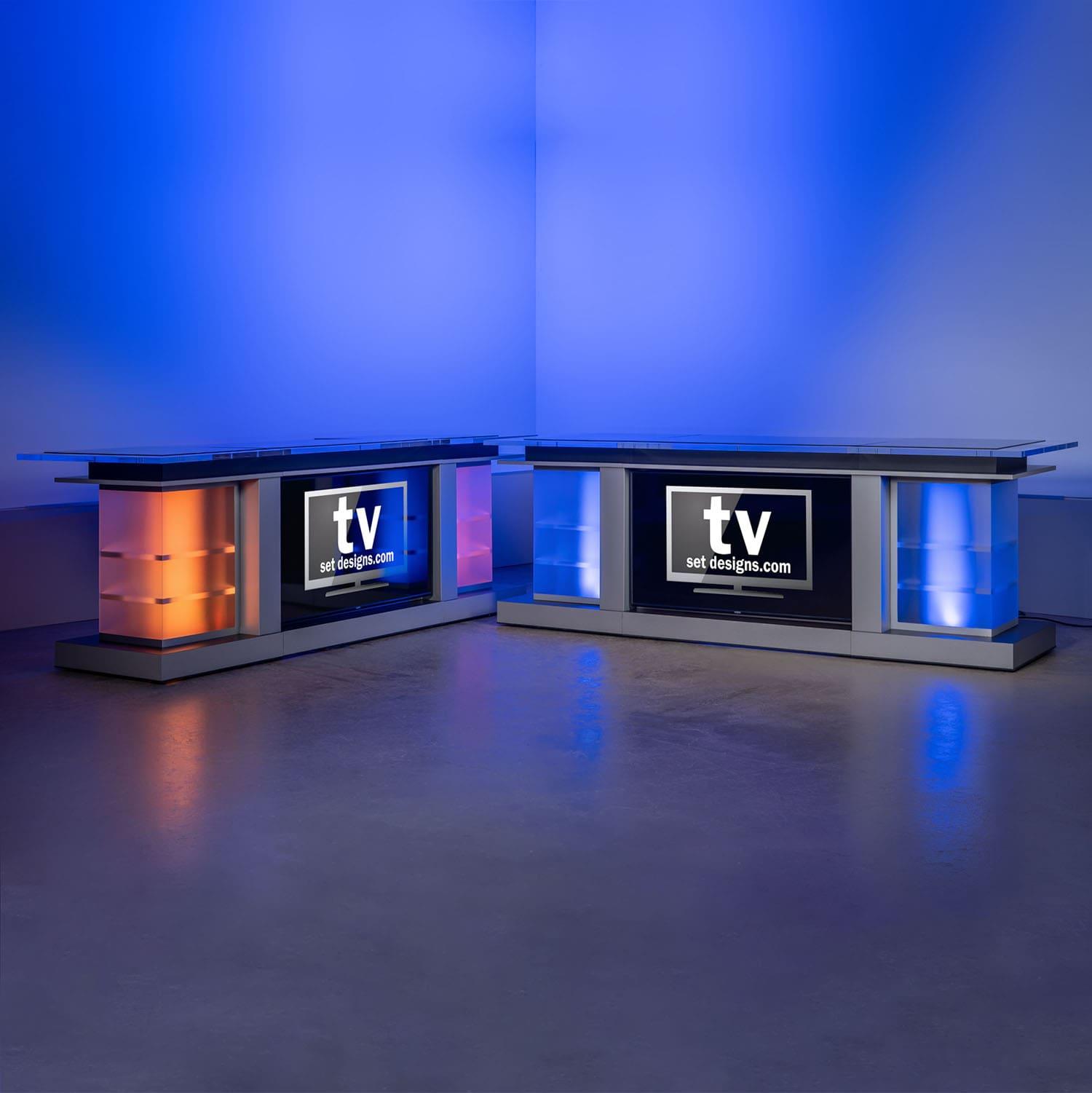This image depicts a photograph of a modern, stylish room characterized by its vibrant blue walls, which exhibit a slightly reflective or possibly translucent quality. The floor is a sleek, polished gray surface that resembles concrete. Positioned diagonally within the room are two distinctive tables, each designed with metallic bases and semi-transparent glass tops and sides. These tables form a four-beaded L-shape structure and are accentuated by a captivating play of colored lights; the left table glows with orange illumination while the right one radiates blue light. These lights not only enhance the visual appeal of the tables but also reflect onto the floor, creating an interplay of hues that complement the room’s overall aesthetics. Centrally positioned between the tables is a black screen displaying white text that reads "TVsetdesigns.com," suggesting this might be an advertisement.